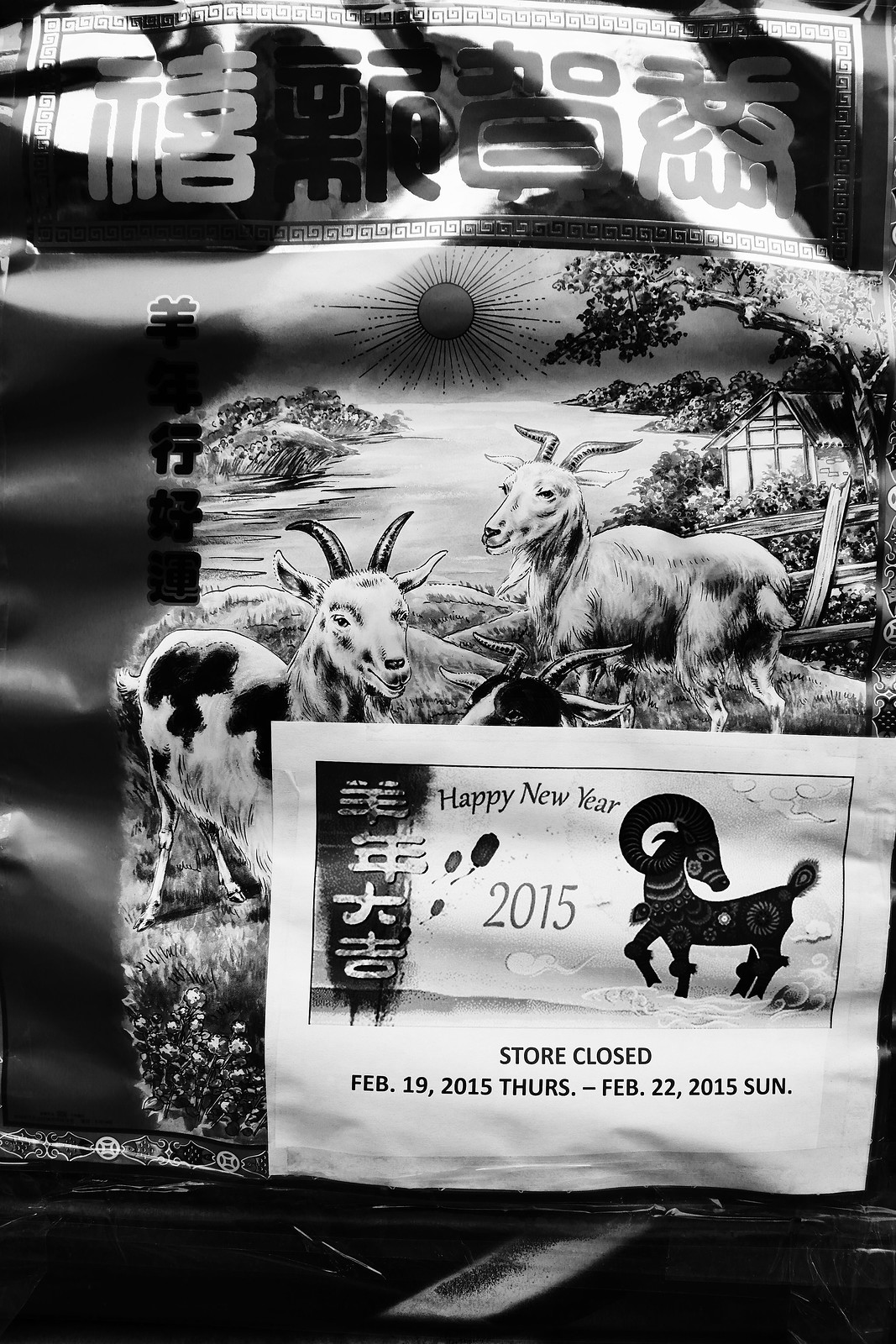This is a tall, black and white poster that appears crinkled and bent, reflecting light at the top. It features an illustration of two large goats standing on a grassy field in front of a wooden fence. One goat is primarily white with large horns, while the other has white fur with black spots and dark horns. To the right of the goats, there is a fence, behind which flowers and a house can be seen. In the distance on the left, a river flows, with wide trees extending over the water and mountains visible in the background. The sky is detailed with the sun at the center, casting long rays. At the very top of the poster, there is a shiny rectangle with four Chinese characters. In the bottom right corner, there is a wide, white piece of paper labeled with text in both a foreign script and English. The English text on the label reads: "Happy New Year 2015. Store Closed February 19, 2015 Thursday - February 22, 2015 Sunday." The background of the entire composition is black.